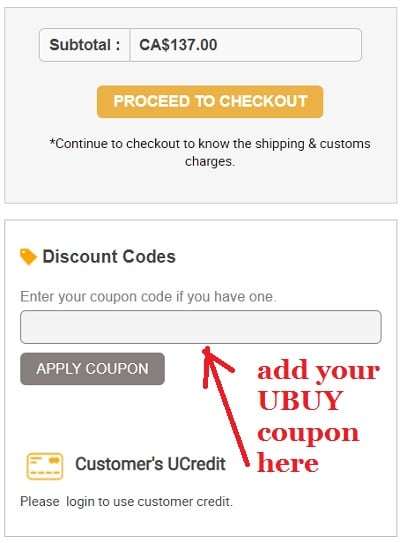Screenshot of a web page displaying the subtotal section of a shopping cart. The top section features a dark gray background. In the center, an off-white rectangle displays bold black text reading "Subtotal" followed by a placeholder for the total amount. To the right, the abbreviation "CA" signifies the state, next to a dollar amount of $137. Below this, an orange and white button prominently invites users to "Proceed to Checkout." A star icon is adjacent to a black text note that states, "Continue to checkout to know the shipping and customs charges."

The background of this section appears in mid-gray. An orange tag labeled "Discount Codes" is displayed in black text. Below this, gray text prompts users to "enter your code if you have one." A gray rectangle is provided for entering the code, and beneath it, a black rectangle with white text in all caps reads "APPLY COUPON." A red arrow points to the right side of the section, where red text instructs users to "add your Ubuy coupon here."

Further down, an orange credit card icon is displayed beside black text that reads "Customers Ucredit." Below this, smaller black text advises, "Please log in to use customer credit." This entire section is bordered in black.